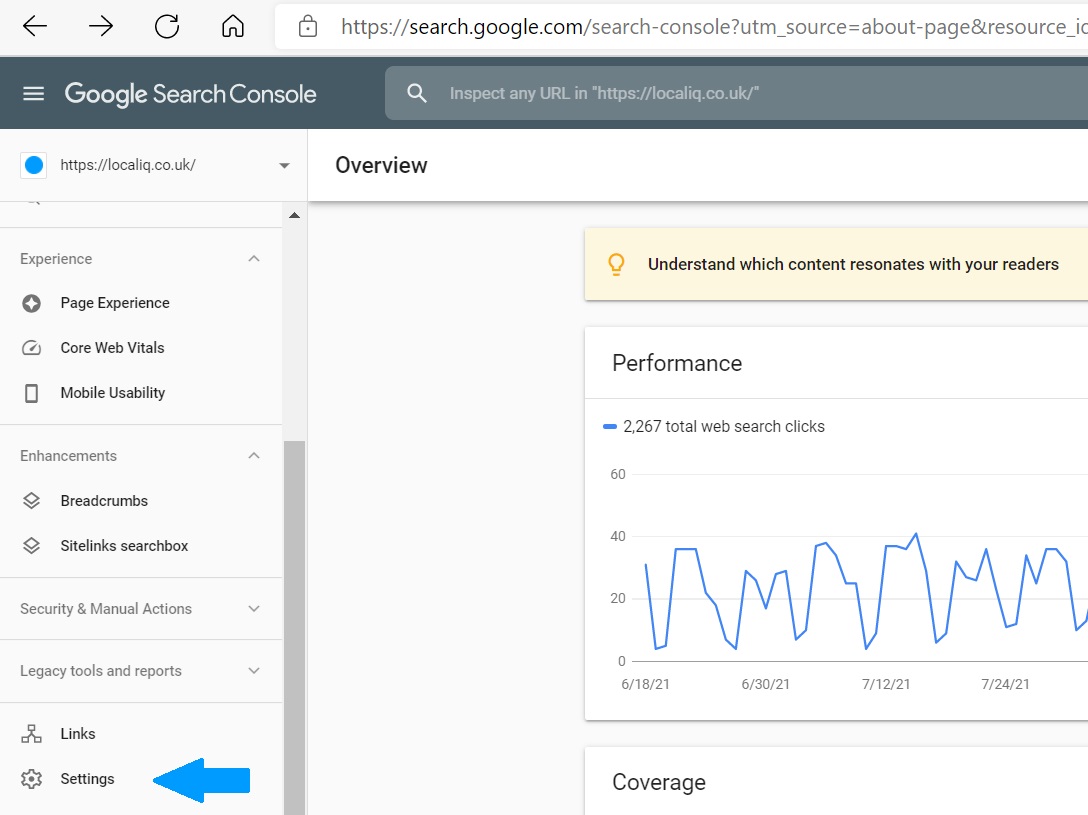This is a detailed screen capture of the Google Search Console interface. At the top, there's a gray navigation bar featuring a black back arrow, a black forward arrow, a refresh button, and a home button. The address bar below it is white with a padlock icon, indicating a secure connection, and displays the URL: "search.google.com/search-console."

Beneath this, another gray bar displays the heading "Google Search Console" with a hamburger menu icon (three horizontal lines) to the left. Below it is a gray input box that reads "Inspect any URL" with a URL, "https://localiq.co.uk," entered within.

To one side, the interface has a white submenu featuring "localiq.co.uk" with a blue and white circle icon beside it. The submenu is surrounded by various gray icons and texts, including "Experience" and "Page Experience" with a star icon, "Core Web Vitals" with a cloud icon, "Mobile Usability" with a cell phone icon, and "Enhancements," which lists "Breadcrumbs" and "Sitelinks search box," each accompanied by small square icons.

Further down, there are sections labeled "Security and Manual Actions" and "Legacy Tools and Reports," each with a down arrow for expanding options, "Links" with an interconnected blocks logo, and "Settings," marked with a cogwheel icon and highlighted by a blue arrow pointing at it.

On the other side of the image, the top section is labeled "Overview" in black. Below this, a yellow box with a lightbulb icon reads "Understand which content resonates with your readers." Following this, there is a performance chart displaying "2,267 total web search clicks" in blue and black text, with data ranging from June 18, 2021, through July 24, 2021, illustrated by a blue line graph. At the bottom of this section is the heading "Coverage."